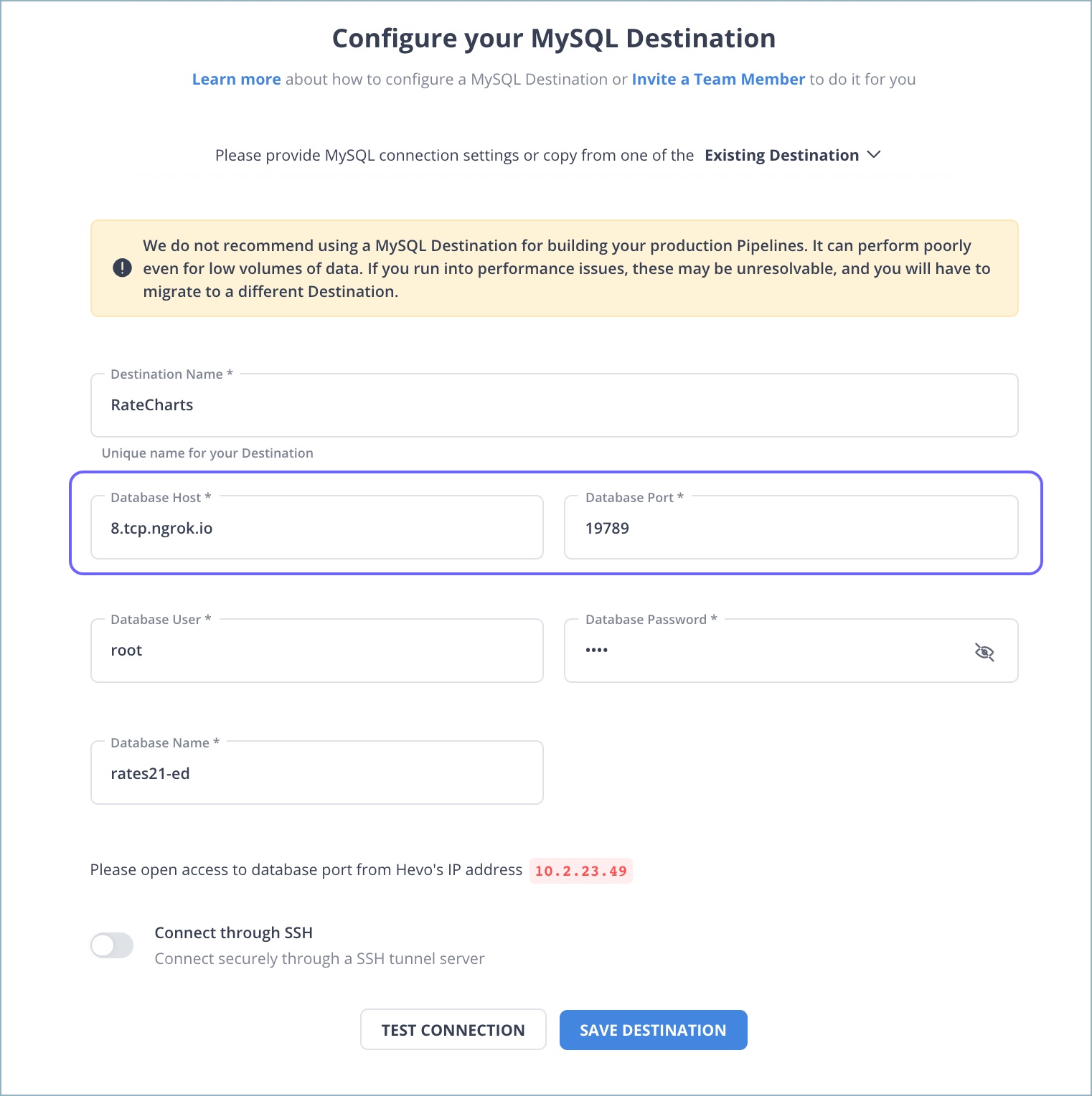A detailed descriptive caption:

In this manual screenshot, designed to guide the user through configuring a MySQL destination, the page prominently features a blue outline and a white background. The predominant colors are white, black, blue, and tan, giving the page a clean, professional look.

At the top, a heading in bold black sans-serif font reads "Configure Your MySQL Destination." Beneath this, a smaller text instructs users on how to configure the MySQL destination or invite a team member for assistance, with "learn more" and "invite a team member" appearing as bolded blue hyperlinks.

A noticeable tan callout box below provides a critical warning: "We do not recommend using a MySQL destination for building your production pipelines. It can perform poorly even for low volumes of data. If you run into performance issues, these may be unresolvable, and you will have to migrate to a different destination." This text is also bolded, emphasizing the importance of the caution.

The page then transitions into step-by-step field entries essential for creating new destinations. It includes labels and fields for "Destination Name," "Destination Host," and "Database Port," with particular fields highlighted to direct user focus.

At the bottom of the page, two clickable buttons labeled "Test Connection" and "Save Destination" provide users with actionable options to validate their input or save their settings.